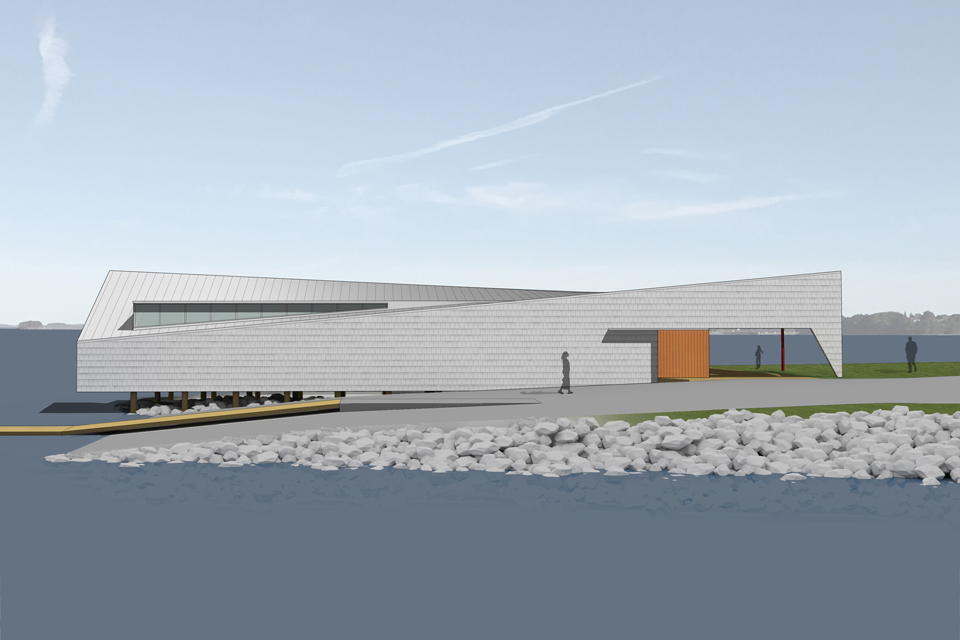This horizontally oriented, digitally rendered image depicts a modern, postmodern building situated on a peninsula by the water. The building features clean edges and a smooth style, resembling a 3D graphic design. Set against a backdrop of a light blue sky with scattered white clouds, the scene is bathed in daylight.

In the foreground, blue, slightly grayish water forms a C-shape around the land. The coastline is lined with white rocks and stretches of green grass. A gray pavement seems to slope down into the water, resembling a boat ramp, accentuated by a yellow warning stripe.

The building itself is a long, irregularly shaped rectangle with an angled, sloping roof, evoking a design reminiscent of Frank Lloyd Wright's architectural style. The structure is primarily gray with white vertical stripes, and an orange wall stands prominently on the right side. Part of the building extends over the water, supported by wooden posts. The left section of the building features minimal windows, while a small elevated section above the slanted roof contains additional windows, creating a unique, visually appealing profile.

Three gray, shadowy silhouettes of people are dispersed around the building: one figure in a dress is walking, another stands beyond the entrance overhang, and a third figure is present in the grassy area in front of the building.